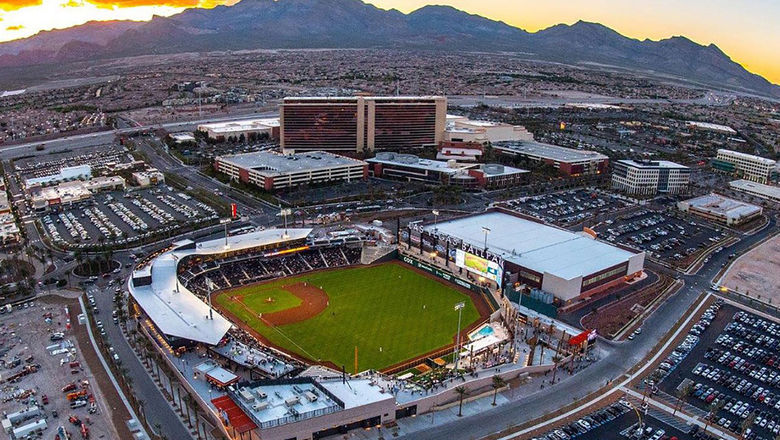This aerial image captures an expansive and vibrant vista of a city with a central focus on a bustling baseball stadium, identified by the sign "Las Vegas Ballpark". Taken either from an airplane or a blimp, the view provides a bird’s-eye perspective, showcasing the lush green grass and distinct brown infield areas where bases are located, with stadium seating filled with spectators and visible players on the field, indicating a game in progress. Encircling the stadium are large parking lots teeming with cars, hinting at the event's popularity. Beyond the immediate vicinity, an array of buildings, shopping areas, and hotels populate the scene, with numerous roads and highways crisscrossing through the landscape, connecting different parts of the city. On the horizon, the city skyline features prominently, with notable tall buildings, including one with striking glass windows. Further behind, a neighborhood of houses stretches toward distant mountains, which frame the stunning orange hues of a sunset peeking through the top left corner and casting a beautiful glow over the scene, signifying the transition from day into evening. This detailed and dynamic photo captures both the energy of the baseball game and the serene beauty of the natural landscape in the backdrop.